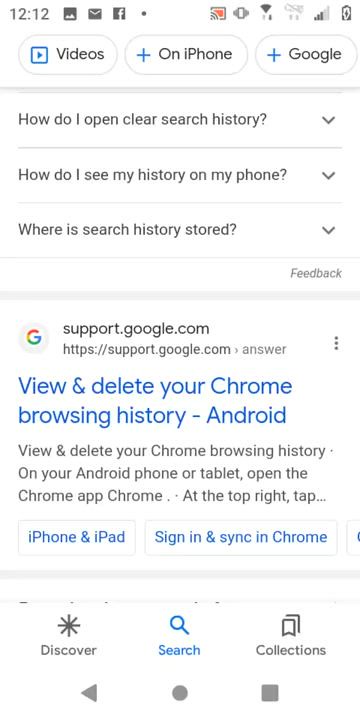This screenshot, captured from an Android mobile phone, showcases several elements of a user interface in a vertically-oriented, rectangular format. The status bar at the top indicates the time as 12:12, accompanied by an envelope icon, suggesting an unread email, and the Facebook app icon. To the far right, the signal strength is displayed with three out of five bars, a Wi-Fi signal icon, and a battery percentage indicator showing the power level.

Below the status bar, there is a search query area displaying various questions such as "How do I open clear search history?", "How do I see my history on my phone?", and "Where is my history stored?". The screen also features a blue banner with the word "Videos" and a play button symbolizing video content. Further down, there are options for interacting with the phone, including "On iPhone," a plus sign, and a plus sign with "Google."

At the bottom of the screen, the navigation bar includes various function icons: a play button, a record button, a stop button, a discover button marked with a gray asterisk, a search button illustrated by a blue magnifying glass, and a collections button.

Towards the lower part of the screen, there's a link to a Google support page, clearly indicating support.google.com, with a focus on "View and delete your Chrome browsing history." The word "Android" is highlighted in blue, emphasizing that the instructions pertain to Android devices.